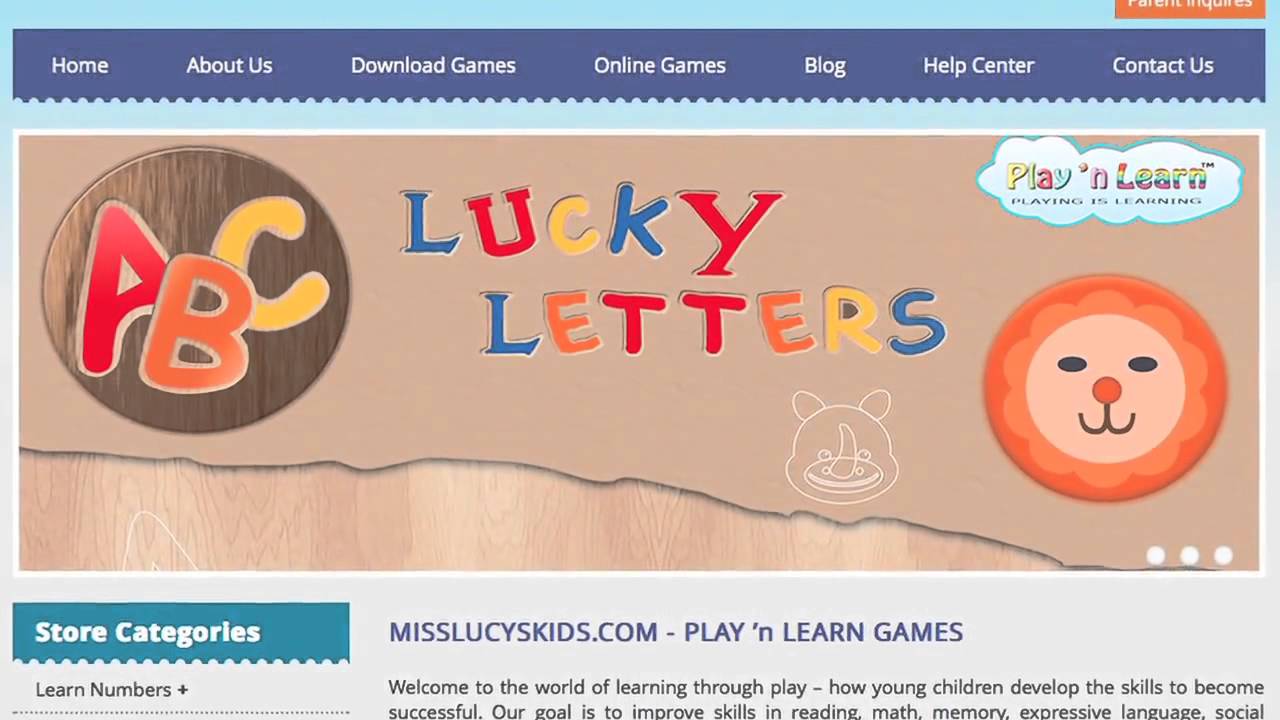Homepage of MissLucyKids.com

The homepage of MissLucyKids.com features a visually captivating and structured layout. At the top, there is a light blue banner. On the top-right corner, partially visible, is a green tab. Directly beneath this, half of the letters spelling “Parent Inquiries” can be seen, yet the text remains discernible.

A purple border spans almost the entire width of the page under the aforementioned section. The left and right sides of the page are adorned with a blue color that shifts to a lighter grayish shade halfway down. In the darker blue areas, approaching a purple hue, white text is displayed. From left to right, the tabs read as follows: "Home," "About Us," "Download Games," "Online Games," "Blog," "Help Center," and finally, on the right, "Contact Us."

A smaller, highlighted number “3” in a blue border is noticeable. Encircling the main content area is a white border. Inside this white border, the background is a tan color. On the left side, there is a large, circular, wooden texture element with a red "A" and a yellow "C" on either side. Overlapping these letters is an orange "B" at the bottom.

Outside this centerpiece, “LUCKY” is spelled out in large, capitalized letters: a blue "L," red "U," yellow "C," blue "K," and red "Y." Beneath this, smaller letters are colored distinctively: orange "E's," red "T's," blue "L" and "S," and a yellow "R." Below this text is the white outline of a rhinoceros.

In the top-left corner, there is a multicolored cloud that reads "Play and Learn," followed by smaller black text stating "Learning is Fun." Below these motivational messages, there is a flower-shaped circle showing a face with black eyes, an orange nose, a "J"-shaped mouth, and three white dots below it.

Towards the bottom-left, beneath the light blue border, there is a dark blue tab with white bold text that says "Store Categories." Below this in black text is "Learn Numbers Plus."

Positioned towards the center, the URL "MissLucyKids.com-playandlearn-games" is prominently displayed in uppercase letters. Directly below this URL, there are two lines of smaller black text providing additional information.